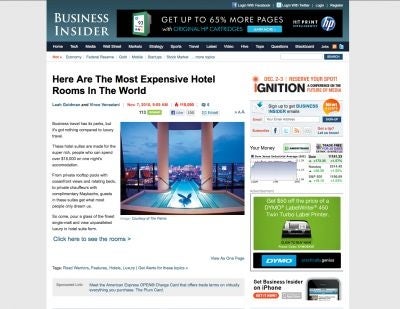Screenshot of a Business Insider article featuring the headline "Here Are the Most Expensive Hotel Rooms in the World." The top of the page displays a distinctive teal banner stretching across the entire width, with the site's name "Business Insider" prominently displayed. Below the header, there's a somewhat blurry advertisement promoting HP digital products, claiming users can get up to 65% more pages, alongside the recognizable HP logo.

The main content area includes a photograph that appears to be of a lavishly designed blue illuminated staircase, though it could also be interpreted as part of a luxurious pool setting. The article itself delves into opulent hotel accommodations globally. Along the right-hand side of the page, there are numerous advertisements, as well as sections that may contain stock market updates and other financial information, enhancing the user experience with diverse content.